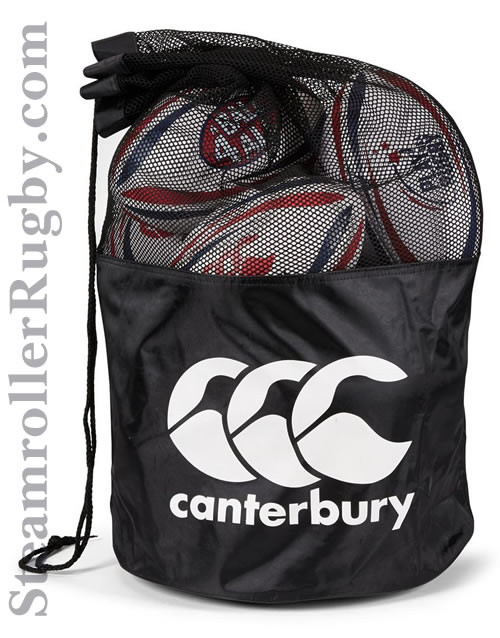The image depicts a black bag with a mesh top, branded with the word "Canterbury" in white lowercase letters. The bag is filled with rugby balls, not footballs, as indicated by the website "steamrollerrugby.com" displayed in light blue text to the left. Inside the bag, which is secured with a black drawstring, there are three visible rugby balls. These balls are predominantly white with red and blue stripy accents and feature various logos and text. One ball has the slogan "play rugby" and another reads "ball for all." The backdrop is white, providing a clear contrast to the black bag and the colorful rugby balls within. The silhouette of a kiwi bird is also visible on the balls, adding a distinctive touch to their design.